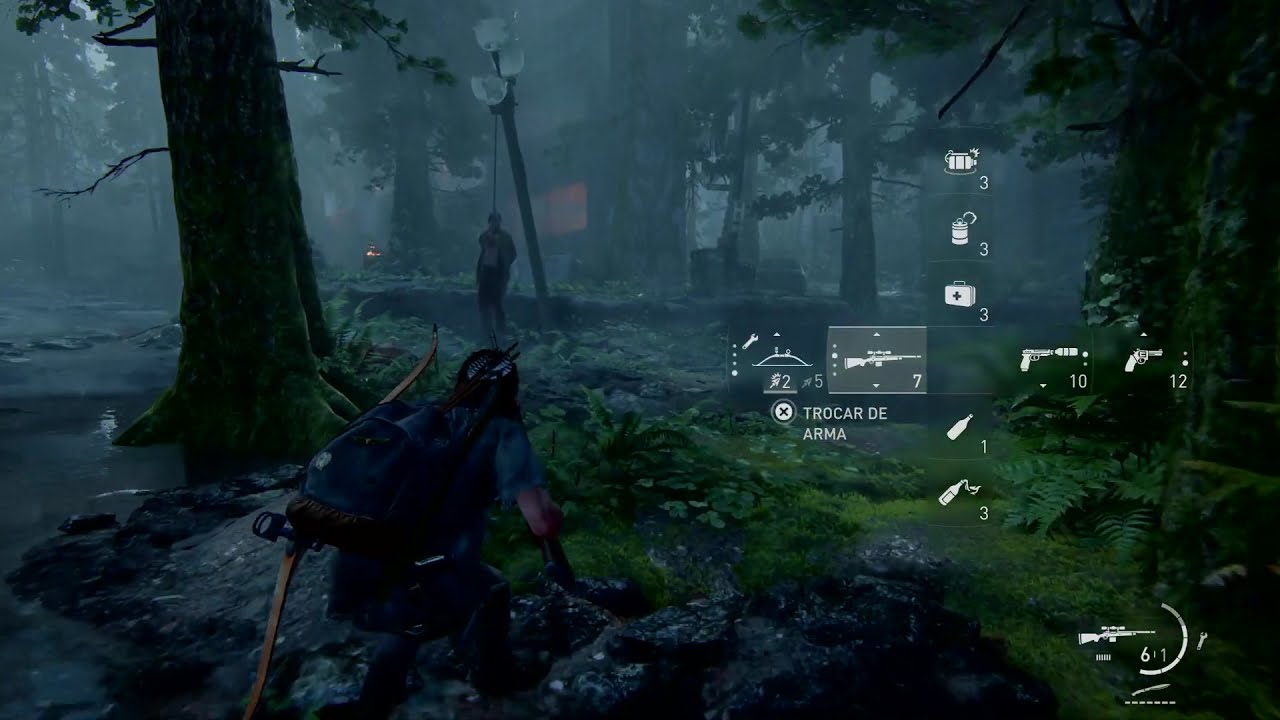In this dark and atmospheric nighttime screenshot from a video game, the setting is a swampy forest area filled with dense green foliage and scattered gray rocks. At the bottom center of the image, a woman is seen walking cautiously through the forest. To her left, a tall tree emerges from a stream, draped in green moss. In the middle foreground, a crouching man with a backpack and a wooden bow, grasping a gun, appears to be on high alert, suggesting a stealth or tactical scenario. Looming in the distance, a man is seen hanging from a light post, adding a chilling element to the scene. The right side of the screen features a menu interface displaying weapon options, ammo counts, and text that reads "trokar de arma," reinforcing the game's combat-oriented mechanics. The image's color palette—gray, black, white, brown, blue, and green—enhances its eerie, immersive atmosphere.